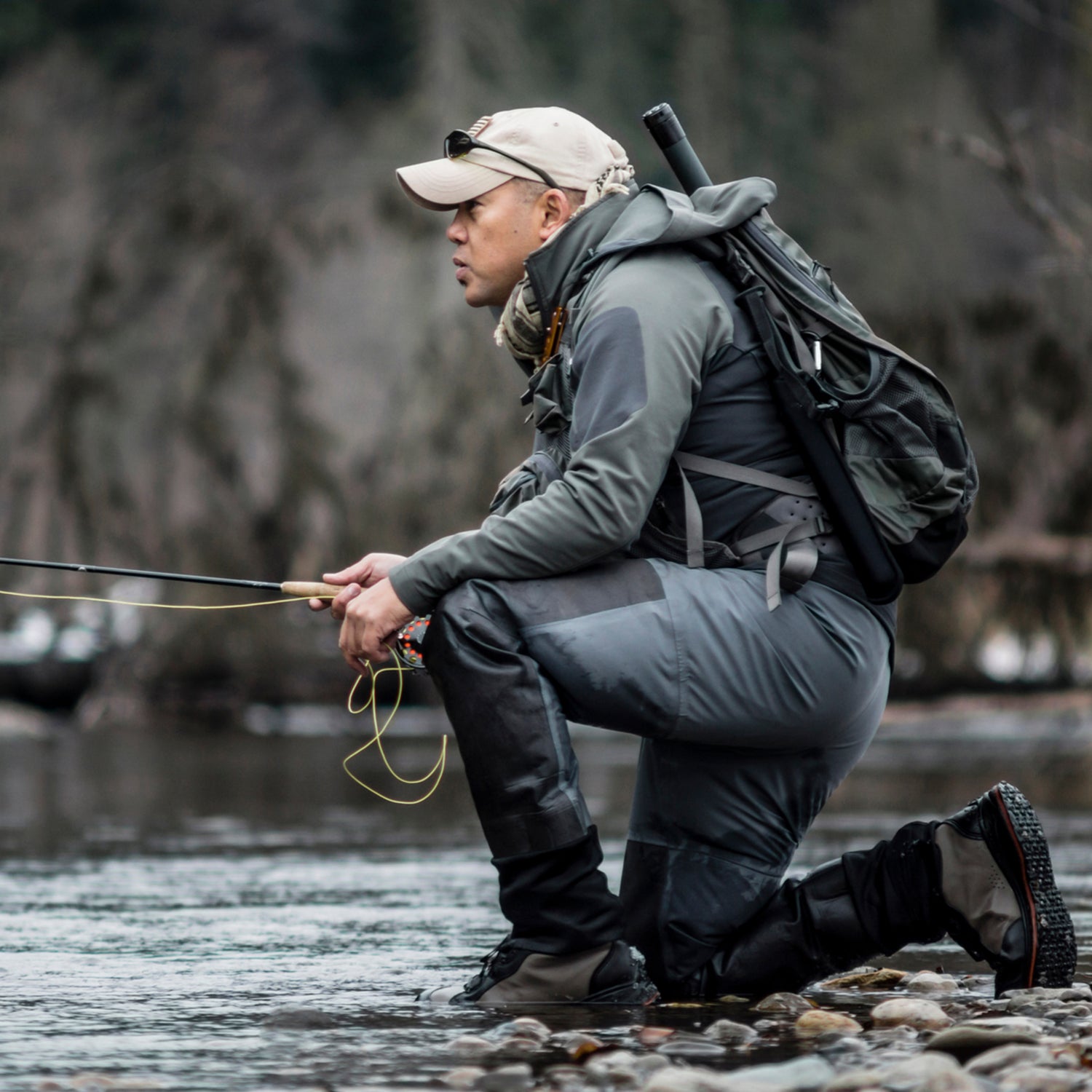In this professional photograph, a man in his 30s is depicted fly fishing by the edge of a creek or river. He is seen kneeling on the rocks, intent on his activity, with a focused and intense expression on his face. The narrow depth of field emphasizes his figure, making the soft, blurred background recede into the distance.

He is outfitted in a dark black and gray sports ensemble, comprised of matching jacket and wader-style pants that appear waterproof. A backpack in a similar dark color scheme is strapped to his back, adorned with various accessories, including what seems to be an umbrella and another rod, possibly a fishing net. His fly fishing rod, held firmly in his hands, features a black graphite-like body with a lighter cork handle, though the tip of the rod remains out of frame.

On his head, he wears a brownish-gray tan baseball cap adorned with an American flag, with sunglasses perched on the bill. The combination of his determined look, reflective sunglasses, and rugged gear gives the image a strong, outdoorsy vibe, suitable for a sportswear advertisement.